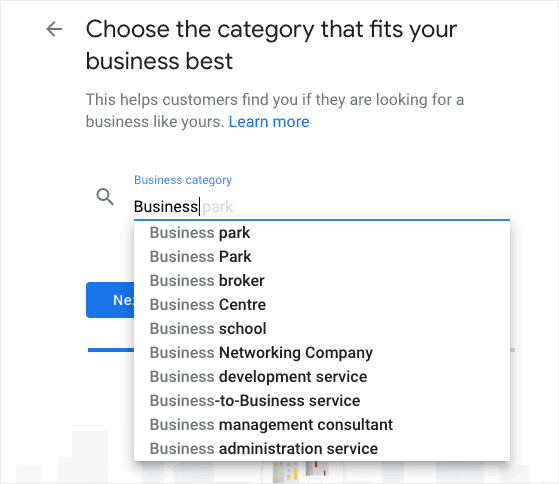The image features a clean white background without any specific indications of its location. Dominating the image is a prominent message in large black font that reads: "Choose the category that fits your business best." Below this, a smaller, gray text states, "This helps customers find you if they are looking for a business like yours." To the right, there is a blue hyperlink labeled "Learn more."

Further down, a search bar is shown with the term "business" typed into it and a drop-down menu displaying various category suggestions. These suggestions include: "Business park," "Business Park" (with a capital 'P'), "Business broker," "Business center," "Business school," "Business networking company," "Business development service," "Business to business service," "Business management consultant," and "Business administration service." The text within the search bar is in gray, while the category suggestions are in black.

Overlaying a section of the form is a "Next" button in blue with white text, along with a horizontal blue line just below it. Part of the lower section of the image contains indistinct visual elements in shades of white, light gray, dark gray, yellow, and red, suggesting the presence of a graphic or illustration of buildings, although the specific details are unclear.

At the top of the drop-down menu is a gray horizontal line, and overall, the content is left-justified. The color palette throughout includes various shades of blue, black, and gray, giving a structured and professional appearance.